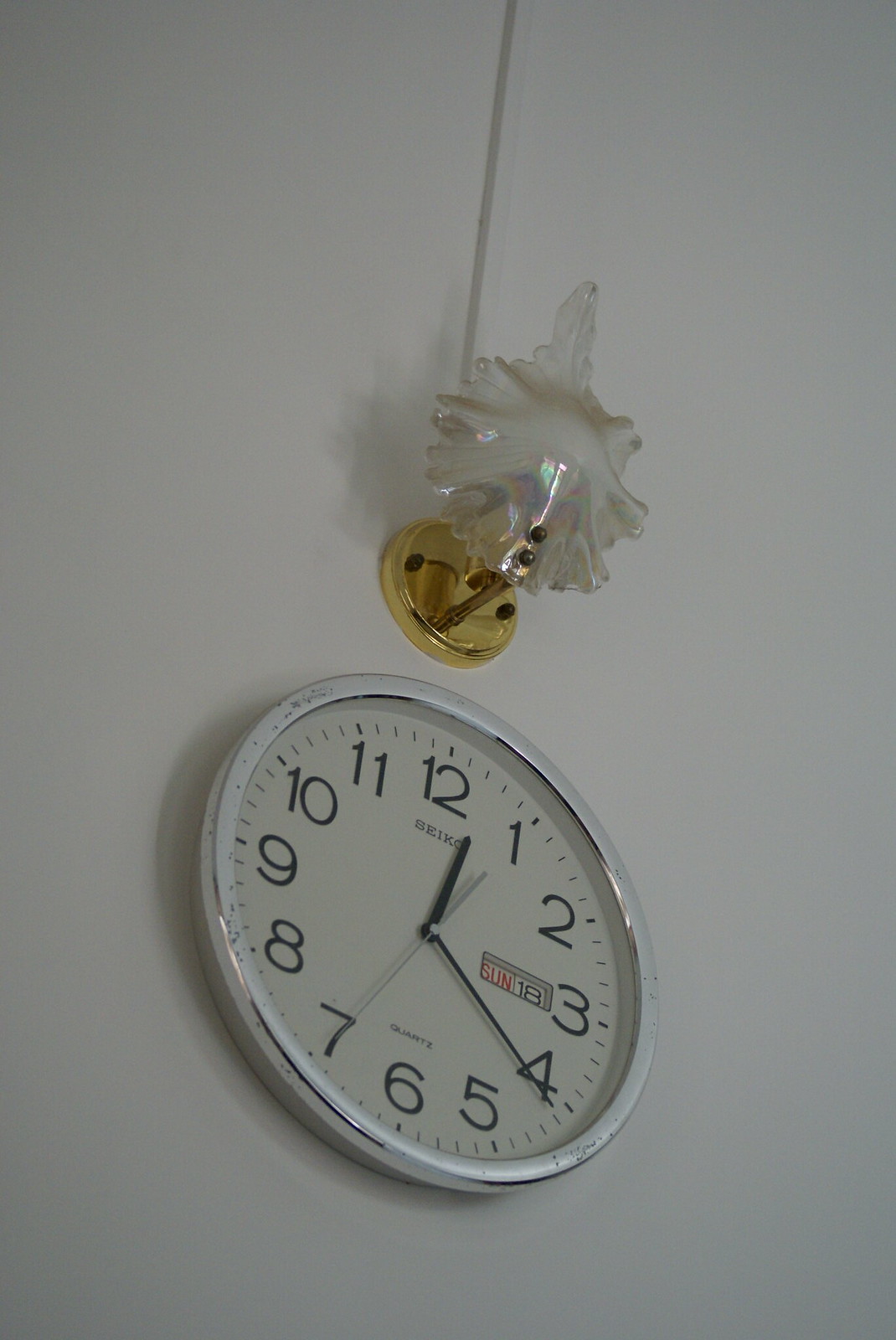A stunning chandelier descends gracefully from the ceiling, resembling a cascade of crystal-clear water droplets splashing onto an object below. This sophisticated fixture is mounted on a gold base, with visible wiring elegantly trailing down from above. Beneath the chandelier, a classic quartz movement clock is prominently displayed. The clock features a white face marked with black numbers in a standard font, and minute markers represented by small black dashes. Encased in a sleek silver chrome frame, the clock also includes a day and date display, currently showing Sunday the 18th. The ensemble of the luxurious chandelier and the timeless clock creates a harmonious blend of elegance and functionality.